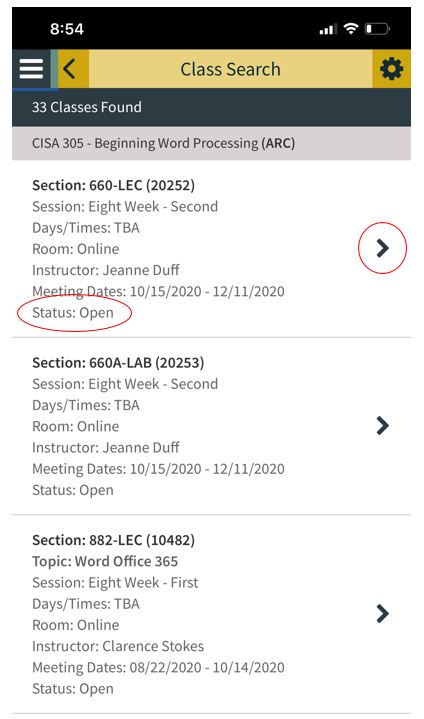The screenshot appears to be from a mobile phone interface. At the top, there is a black status bar displaying the time "8:54" on the left in white, along with mobile icons and a nearly empty battery icon on the right. Below the status bar, there is a yellow header with the text "Class Search" centered. On the left of this header, there is a black left arrow and a "hamburger" menu icon (three horizontal lines), depicted as white on grey with a blue edge. On the right side of this yellow header is a gear icon.

Immediately below the yellow header, there is a grey band with the text "33 classes found" in white. Under this, a lighter grey band has darker black writing that reads "CISA 305 Beginning Word Processing (A or C)". A list of three different class results follows, each separated by thin black horizontal lines.

**First Result:**
- **Section:** 660 (LEC, 20252)
- **Session:** 8 weeks
- **Days:** To be announced
- **Room:** Online
- **Instructor:** Jean Duff
- **Meeting Dates:** 10-15-2020 to 11-12-2020
- **Status:** Open (circled in red)
- A small arrow button to the right is also circled in red.

**Second Result:**
- **Section:** 660A (LAB, 201253)
- **Session:** 8 weeks
- **Days:** To be announced
- **Room:** Online
- **Instructor:** Jean Duff
- **Meeting Dates:** 10-15-2020 to 12-11-2020
- **Status:** Open

**Third Result:**
- **Section:** 802 (LEC, 10482)
- **Topic:** Word Office 365
- **Session:** 8 weeks
- **Days:** To be announced
- **Room:** Online
- **Instructor:** Clarence Stokes
- **Meeting Dates:** 08-22-2020 to 10-14-2020
- **Status:** Open